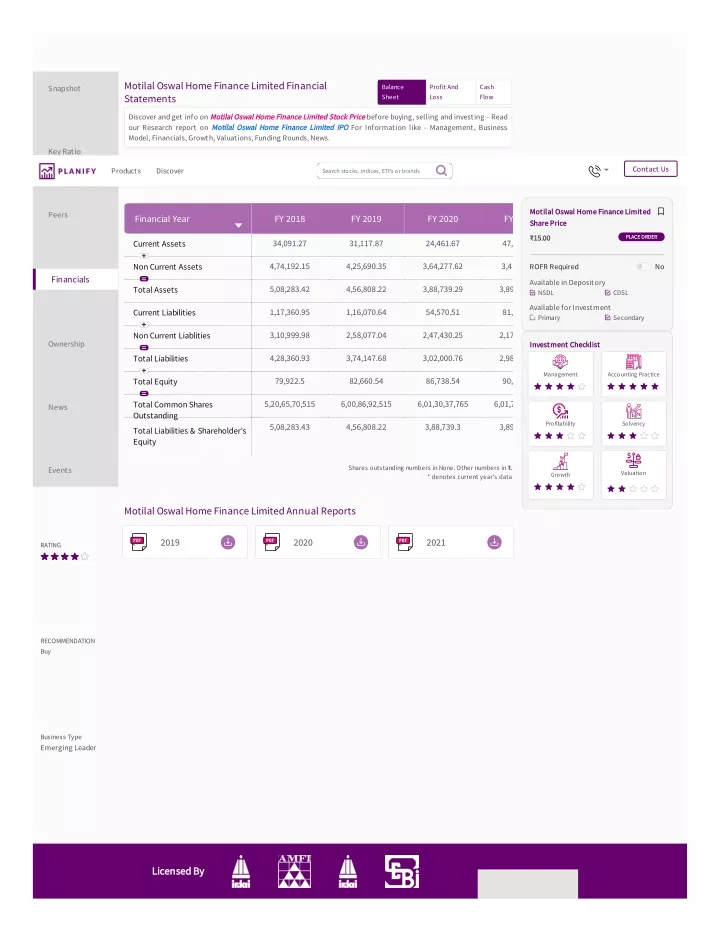The image depicts a financial document page with a complex layout and various color schemes. At the very top, there is a gradient banner that transitions from light purple to dark purple and then to a bluish-purple hue. The central background of the page is white. Prominently displayed at the top is the title "Marital Oswey Home Finance Limited Financial Statements."

On the right side of the title, there's a dark purple rectangular section containing script text. The page's layout includes a column on the left side, which is of average width and colored in a very light lilac. This column is segmented by white spaces. Within these white spaces, there are elements such as a white square featuring a purple label, another white square with purple text, and a rectangular area in light lilac.

Text is organized into columns further down the page. On the far right, there is an additional column that houses some symbols on a white background.

Despite the detailed layout, the text within the document is difficult to decipher, regardless of zooming in or out.